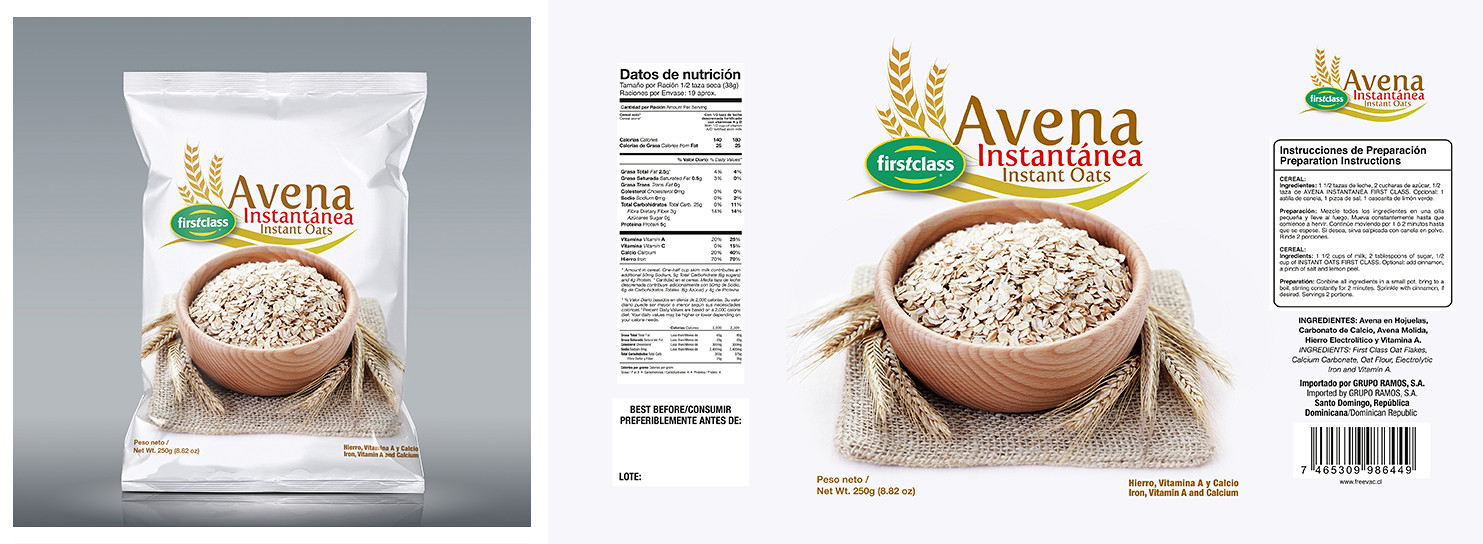This is a side-by-side comparison of two images, showcasing advertisements or packaging for a brand of Instant Oats oatmeal. 

The left image features a rendering of the finished packaging, set against a gray background with dark shading at the bottom to simulate shadows. The package itself is white and prominently displays "Avena Instant Oats" branding. A wooden bowl filled with oats is centrally positioned, adding an appealing, rustic touch to the design. A distinctive green badge labeled "First Class" is prominently placed on the left side of the packaging, emphasizing the high quality of the product.

The right image presents the actual design files for the packaging. The core visual elements, such as the wooden bowl of oats, are consistent with the left image, maintaining the brand's visual identity. However, this image includes additional components that would appear on the back of the finished packaging. On the left section of this design, nutritional details are meticulously laid out, ensuring consumers have access to essential dietary information. The right section provides clear and concise instructions for preparing the oatmeal, contributing to the package's functional and informative nature.